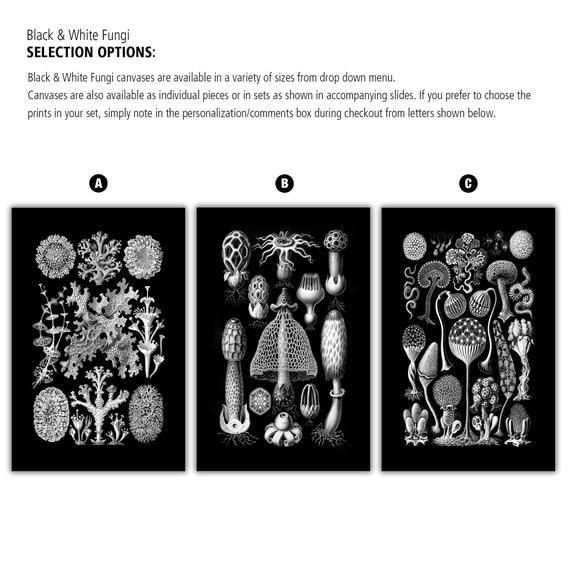The image displays an infographic advertising black and white fungi canvases. It prominently features the heading "Black and White Fungi Selection Options" and explains that these canvases are available in various sizes selectable from a drop-down menu. Customers can purchase them as individual pieces or in curated sets, with the option to personalize their selection by noting their preferences in the comments box at checkout. 

The infographic includes three labeled sections, A, B, and C, each showcasing black canvases with intricate white fungi illustrations. Section A features a composition of four flowers in each corner with additional plant motifs throughout the center. Section B is adorned with a variety of mushroom-like fungi scattered across the canvas. Section C displays an artistic arrangement of flowers, leaves, and mushrooms growing from the bottom upwards. Each canvas is bordered by a one-inch black margin, and the fungi illustrations range from skeletal, see-through designs to more solid forms, capturing the detailed, organic intricacies of the mushrooms and plants.